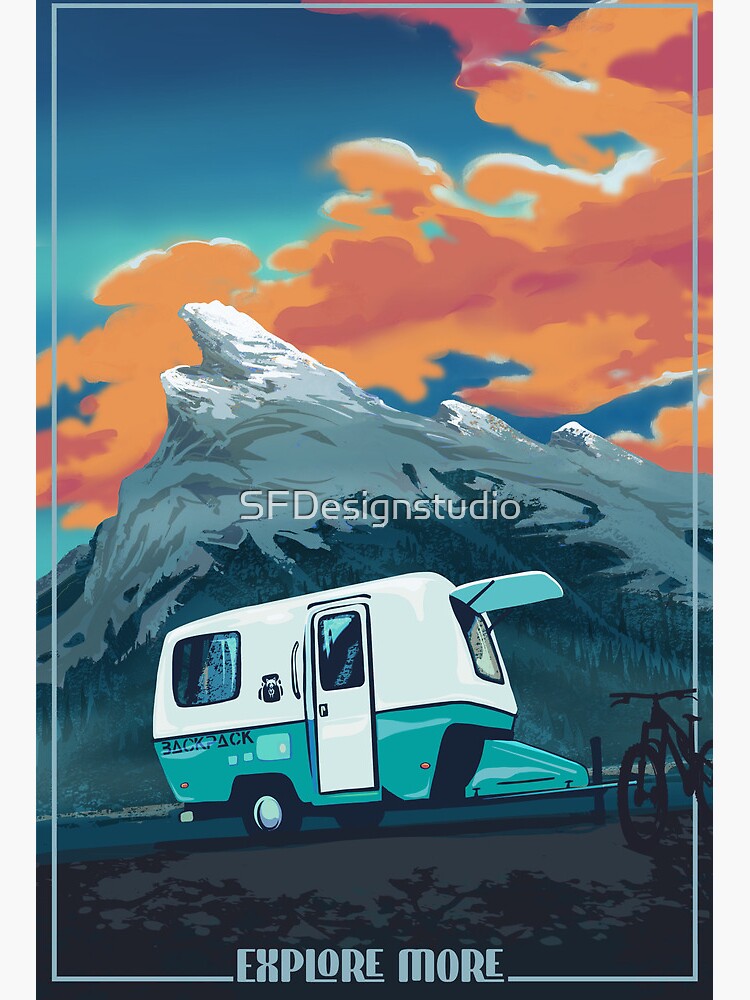This digital artwork, in portrait mode, prominently features a vintage-style camper van that needs to be towed. The camper van is positioned in the lower center of the image and has a white top with a teal green bottom. The van includes a front window propped open, a back window, and a white door with an additional window. The word "BACKPACK" is written on its lower teal section. This camper van is facing right, with the outline of a bicycle in front of it. Above the camper, the text "SF Design Studio" appears in white, while "Explore More" is displayed in a special uppercase font at the bottom. The background showcases a gray mountain with snow-capped peaks, transitioning into an orange-reddish sky, making the scene dramatic and vibrant. The sky also features hints of teal and an orange cloud, giving it a surreal quality. Beneath the bicycle, there are shadows suggesting the presence of trees against the darker foreground.